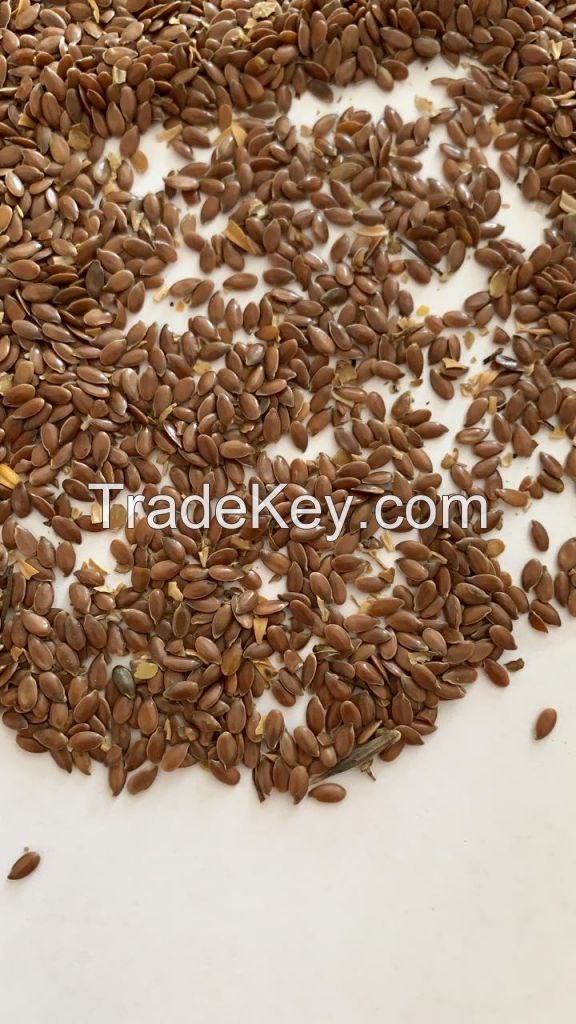In the photograph, a pile of teardrop-shaped flax seeds are scattered across a flat white surface. Predominantly brown, some of the flax seeds exhibit shades of green and dark brown, with a few broken open to reveal a yellow interior. Interspersed within the pile are small yellowish leaf-like flakes. A short green stalk is noticeable near the right side of the image among the seeds. Imposed across the image, in white text with a thin black border, is the website "tradekey.com." The bottom fifth of the photograph displays more of the white surface, with a few stray seeds, one on the left and another on the right. The overall scene gives an impression of an advertisement, with the seeds densely packed at the top and gradually dispersing towards the bottom.